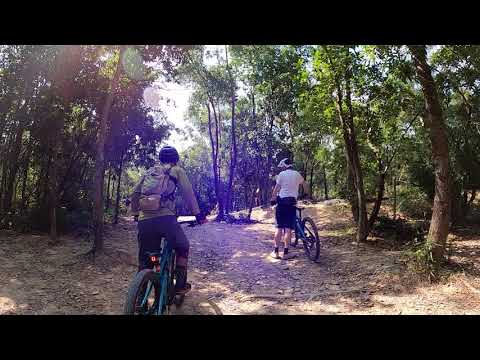The image captures a bright, sunny day in the woods where two bikers are navigating a dirt and leaf-strewn trail lined with trees, indicative of spring or summer. Both riders are wearing helmets and backpacks. The biker in the foreground, wearing a white shirt, black shorts, and a white helmet, is standing beside his bike. Behind him, the second rider, dressed in dark pants and a dark tan or green shirt with a backpack, is pedaling a yellow bike. Shafts of sunlight penetrate the leafy canopy overhead, casting dappled light onto the trail. The trail itself lacks distinct markings, blending seamlessly into the natural undergrowth, yet appears well-traveled with no trees obstructing the path. The scene's composition is framed by a horizontal black bar along the top and bottom.